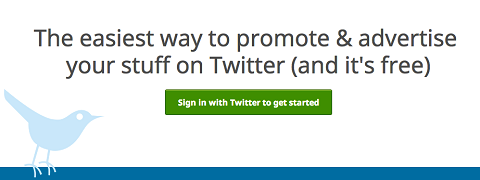The image features a promotional graphic centered around using Twitter as a marketing tool. At the top, there is a dark gray or black text that reads, "The easiest way to promote and advertise your stuff on Twitter (and it's free)." This text is displayed in a basic sans-serif font with a moderately bold appearance, neither fully bold nor entirely regular.

Below the text, a long, slightly dark olive green rectangle is prominently featured, shadowed by a black border. In bold, white lettering within the rectangle, it declares, "Sign in with Twitter to get started."

Towards the bottom left corner of the image, an old-school blue Twitter bird logo is visible. This bird has a simplistic, clip-art style design, featuring a white eye and tail feathers that curve upwards. The bird's design lacks detailed individual feather lines, presenting a more basic and iconic look.

The bird is perched on a long, dark blue divider, with its two front toes or talons extending over the edge. Notably, the bird's beak is very thin and tilts slightly upwards. Positioned as if looking at the viewer from its right side, the bird's beak aligns with the text inside the olive green rectangle.